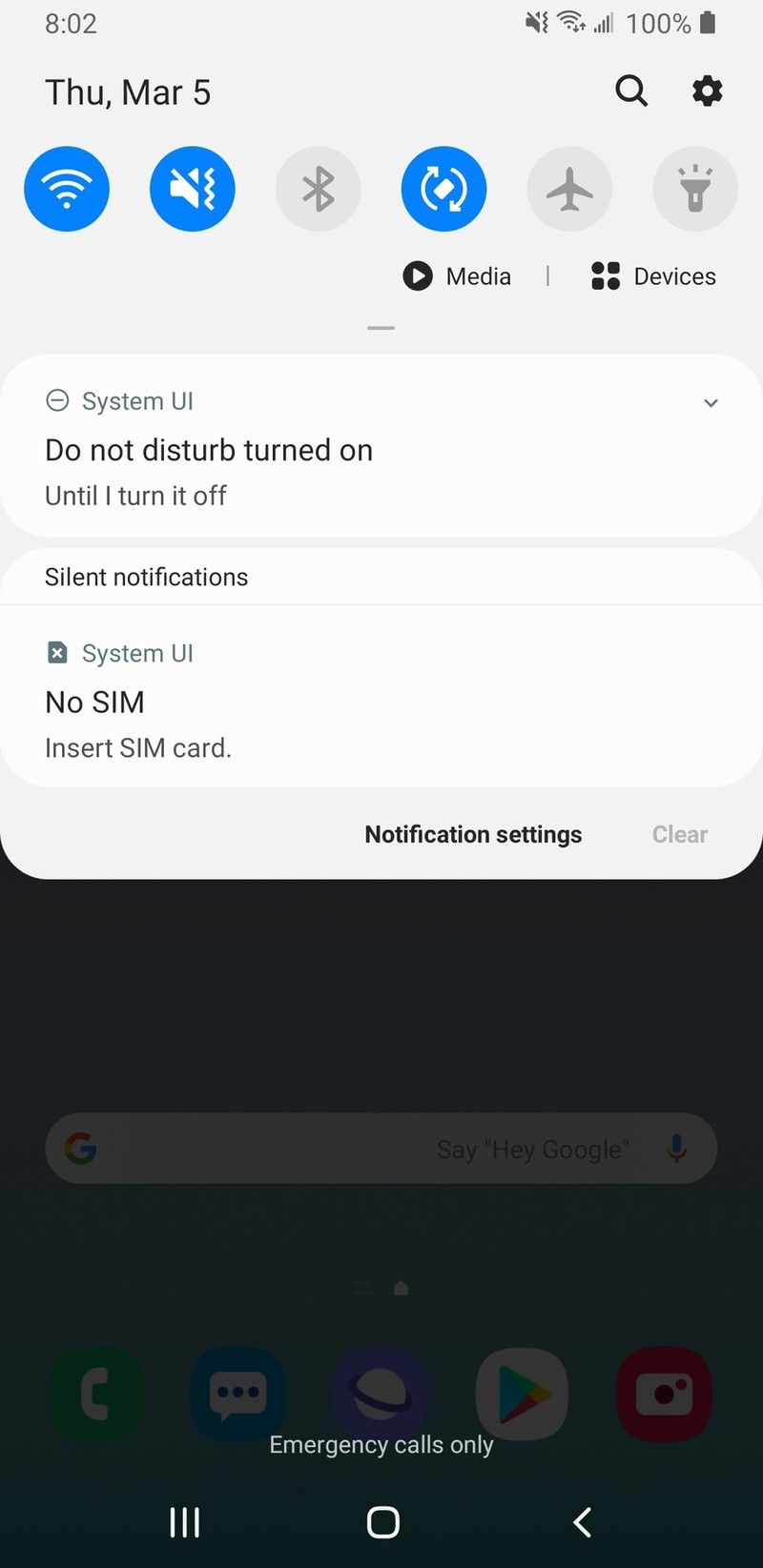The image on the cell phone screen shows a fully charged battery at 100%. The current time reads 8:02, and it is Thursday, March 5th. The top of the screen includes several icons: a search icon, a settings icon, a blue icon indicating loudness, an icon showing there is no ringer, an internet connection icon, an airplane mode icon, an icon with two half circles, a flashlight icon, a media icon depicted as a black circle with a white arrow, and four black dots denoting connected devices. Below this, a notification states "Do Not Disturb is on until you turn it off," and another notification mentions "System UI: No SIM, insert SIM card."

Further down the screen, under a bold "Notification Settings" title, there is a "Clear" button. The lower half of the screen, which is slightly grayed out, features a search prompt saying "Say Google, Say Hey Google," and a notification stating "Emergency calls only," indicating limited call functionality. Behind this prompt, several icons are present but are grayed out and not easily identifiable.